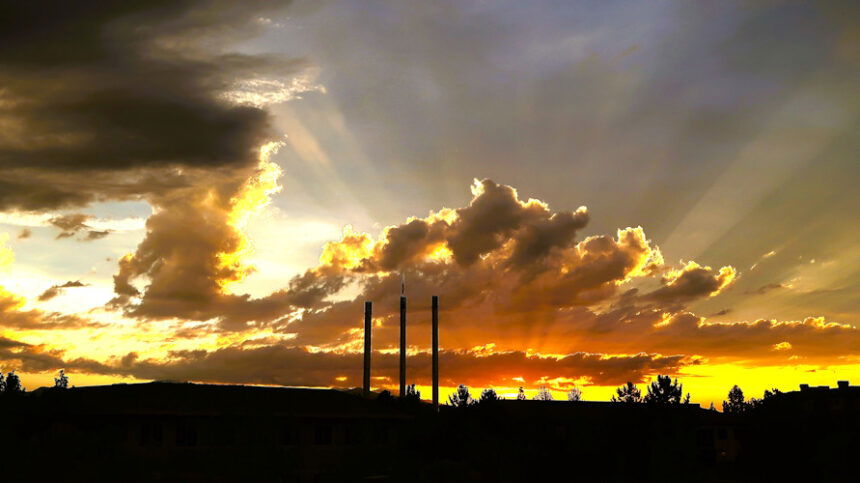In this photograph, an enchanting sunset sky dominates over an industrial landscape, graced with dramatic hues and intricate details. The lower third of the image reveals a blackened landscape, shrouded in shadow, featuring three smokestacks at the center, with faint silhouettes of trees and perhaps even a structural outline, hinting at buildings or houses. The horizon glows with a beautiful golden yellow, transitioning through layers of orange, darkening to purple, and finally blending into the blue of the sky. Above, large billowing clouds, along with darker, more ominous clouds in the upper left, diffuse the sunlight, allowing rays to pierce through and illuminate the scene with striking contrast. Smoke from the chimneys merges seamlessly with the clouds, creating a hauntingly beautiful yet poignant reminder of the landscape's industrial nature.